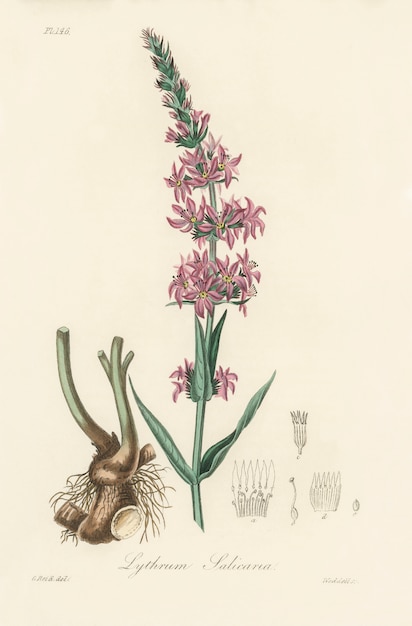The image features a vintage botanical drawing of a plant on an off-white, manila-tinted background. At its base, the plant displays a brown, bulbous root with fine root hairs emerging from its main branches. This root appears on the left side of the image, not planted but vivid against the plain background. The central stem is a light to dark green, rising from the root with a series of leaves and delicate pink flowers featuring yellow centers arranged in rows along the stalk. The plant culminates in a fluffy, green and pink apex, with some flowers just beginning to emerge. Smaller, pencil-drawn illustrations, possibly of the plant’s anatomical details such as its pistils, are situated on the right side of the image beneath the leaves. At the bottom, a cursive inscription identifies the plant as "Lithrum" with varying species names suggested such as "salivarede," "salicana," or "selenia," emphasizing its botanical identity.